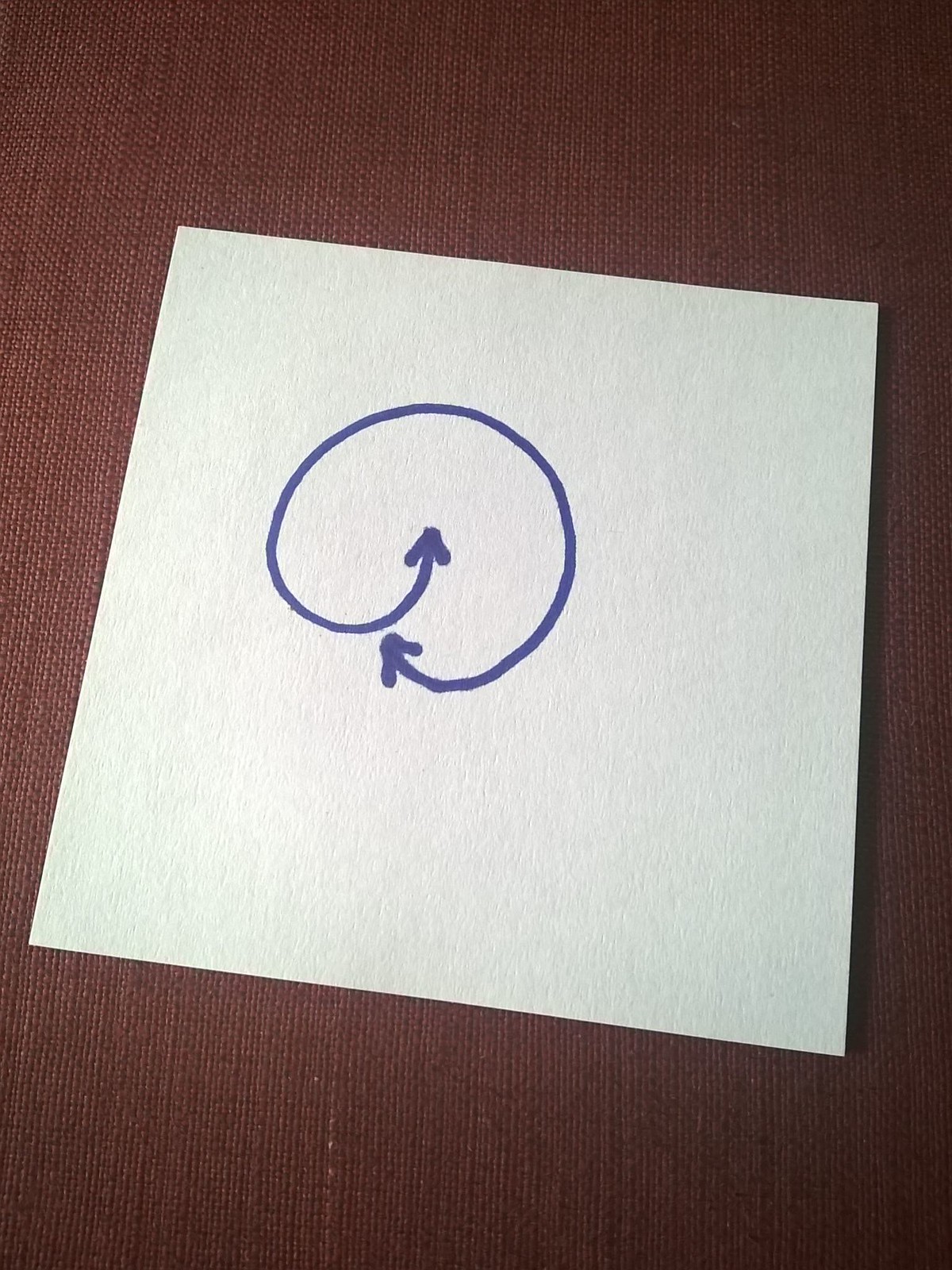A square piece of white textured paper is resting on a brown fabric couch, which is clearly visible in the background with distinct stitch markings. The drawing, created with a blue marker, features an upward-pointing arrow that flows into a curlicue, almost forming a complete circle that loops back to the starting point of the arrow. Notably, dark ink spots mark the ends and curved points of the arrow, suggesting where the marker was pressed down more heavily.